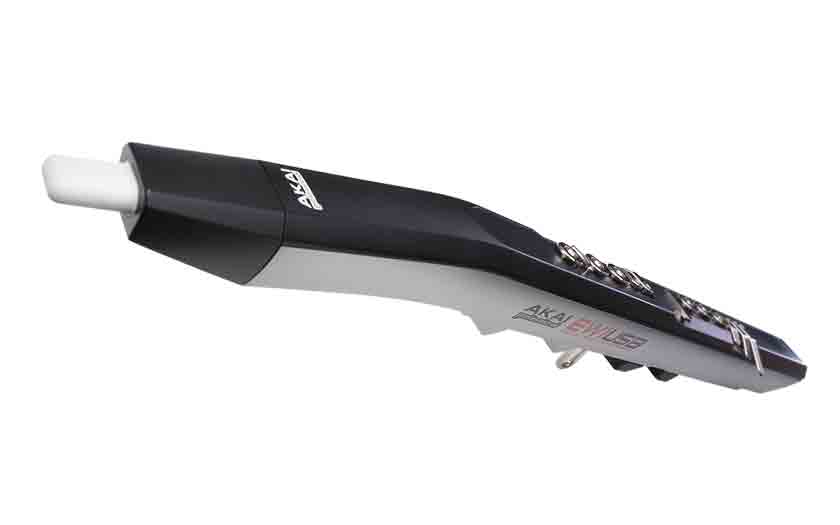This is a photograph of an electronic wind instrument, likely an Akai EWI (Electronic Wind Instrument). The sleek, monochromatic device features a predominantly black body with a frosted white lower section. The instrument has a white mouthpiece on the left and a distinctive black and white handle. The Akai branding "A-K-A-I" is prominently displayed in white lettering on the top of the device, while the side features additional branding with "A-K-A-I" in black and red, followed by the model designation "EWI" printed in black. The device is adorned with an array of keys and buttons, including silver buttons on the top, suggesting its ability to mimic various wind instrument sounds such as a trumpet or saxophone. Its compact, approximately two to three-foot-long form, along with its 80s or 90s design aesthetic, makes it stand out as an innovative and versatile electronic instrument.